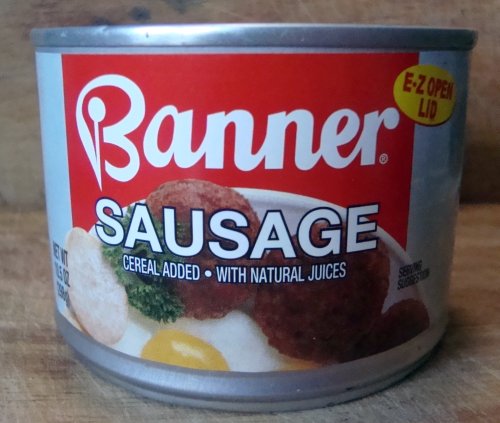The image showcases a silver can of Banner Sausage, prominently placed on a light-colored wooden table with a matching light brown background. The can features a distinct red and white label. In bold white text against the red section, the brand name "Banner" is clearly visible. A small yellow oval above the brand name highlights an 'Easy Open Lid' feature. The label also includes a graphic depiction of a breakfast plate, complete with a sunny-side-up egg, sausage links, a biscuit, and greens, possibly kale. Notably, the label indicates "cereal added with natural juices," creating an unusual combination for a sausage product.